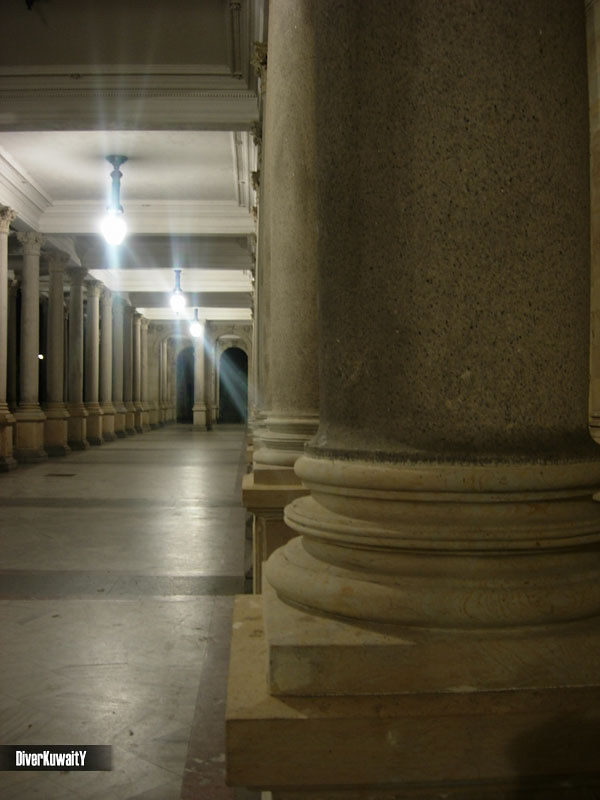This image depicts an exterior stone corridor with a series of light to medium brown pillars running along both sides, indicative of weathered exposure. The corridor, presumably from an older-fashioned building, features intricately designed columns with ornate details at both the base and top. Three illuminated white bulbs hang from the ceiling, casting light along the walkway in a pattern that appears to coincide with the segmented stone floor, which exhibits varying lighter and darker elements divided by gray lines. In the distance, the corridor culminates in two dark archways flanked by additional pillars, inviting further passage but shrouded in shadow, suggesting that the photograph was taken at night. The overall composition highlights the symmetry and architectural elegance of the scene.